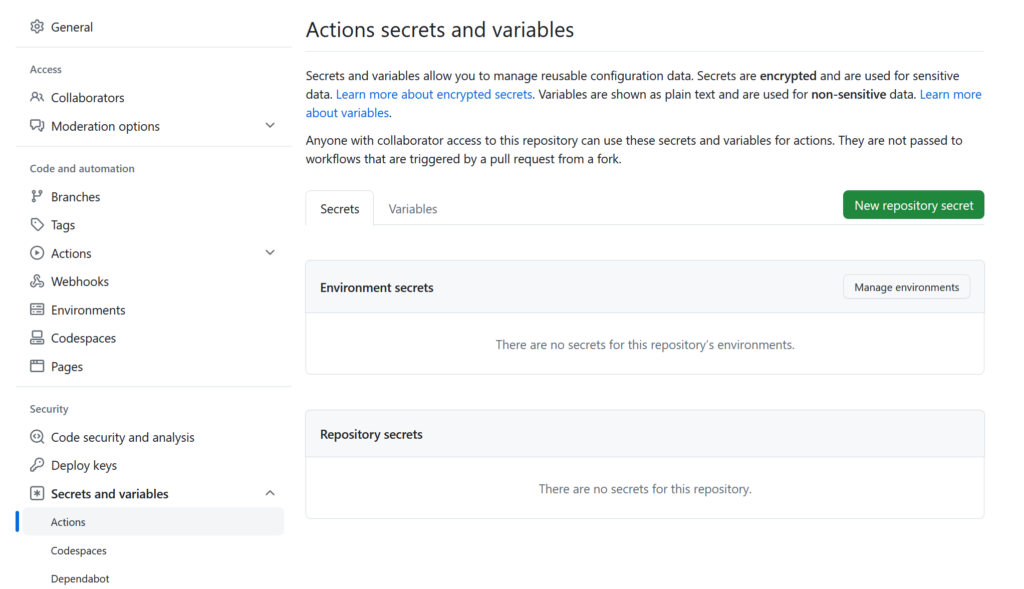Screenshot depicting a two-column layout interface in landscape mode, likely from a settings dashboard.

In the left column, the upper left corner features a "Settings" header followed by a "General Settings" icon. Below it, separated by a gray line, are multiple sections and options: "Access," "Collaborators," "Moderation Options" with a drop-down menu, followed by another gray line. Next is the "Code and Automation" section, listed with the following rows, each accompanied by icons: "Branches," "Tags," "Actions" (with a drop-down menu), "Webhooks," "Environments," "Codespaces," and "Pages." Following another gray line, the next section is "Security," which includes "Code Security and Analysis," "Deploy Keys," and a bolded "Secrets and Variables," which has an up arrow indicating that this menu is expanded. The row "Actions" is highlighted in gray with a blue line adjacent to it and is connected to the "Codespaces" and "Dependabot."

In the upper right-hand corner of the second column, under the "Actions" of the "Secrets and Variables" section, text explains, "Secrets and variables allow you to manage reusable configuration data. Secrets are encrypted and used for sensitive data," followed by a blue hyperlink text saying, "Learn more about encrypted secrets." Further down, it mentions, "Variables are shown as plain text and are used for non-sensitive data," with another blue hyperlink text, "Learn more about variables." Below these descriptions are two tabs, "Secrets" and "Variables." 

A prominent green button labeled "New Repository Secret" is located beneath them. The next section is titled "Environment Secrets," and at the end, there is a button labeled "Manage Environments."